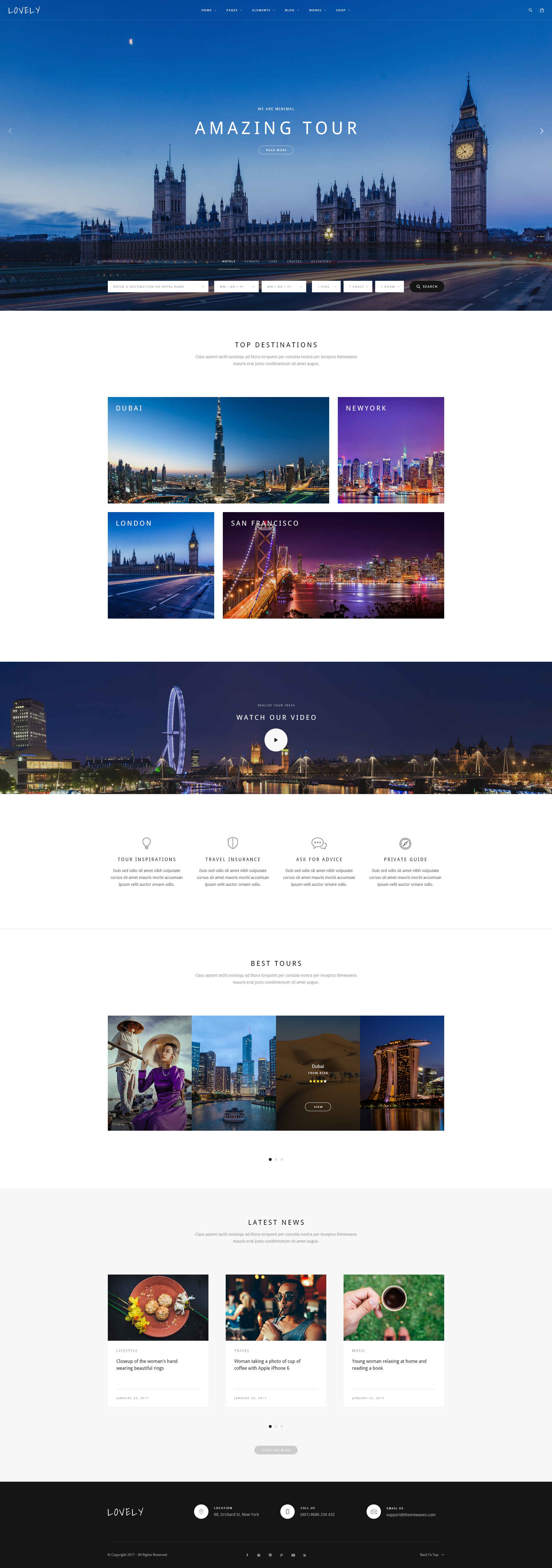The image appears to be a detailed travel advertisement showcasing top destinations across the world.

At the top, it features the word "Lovely" prominently, though the smaller print is hard to decipher completely. The larger text beneath reads, "Amazing Tour." The main visual elements are as follows:

- **Top Picture:** A stunning night-time cityscape of Dubai, illuminated beautifully with glittering lights.
- **Beside Dubai:** The iconic New York City skyline, painted in hues of blue, purple, and light pink, with the Hudson River shimmering in the reflective city lights.
- **Bottom Left:** A classic image of London, featuring the grand and historic clock tower (likely Big Ben) with a road stretching ahead.
- **Beside London:** The picturesque Golden Gate Bridge in San Francisco, lit by the city's night lights and reflected in the surrounding water.

Underneath these primary images, the caption reads "Watch Our Video," accompanied by an image of a giant Ferris wheel and a cityscape against the night-time sky, illustrating vibrant urban lights.

Another section labeled "Best Tours" features an image of a woman on a boat, followed by several more captivating cityscape pictures, highlighting the appeal of nighttime glimpses of Dubai once more.

The "Latest News" section includes diverse visuals:
- A scrumptious display of food,
- A person possibly playing a musical instrument,
- Lastly, an individual engrossed in reading something, set against a backdrop of grass or greenery.